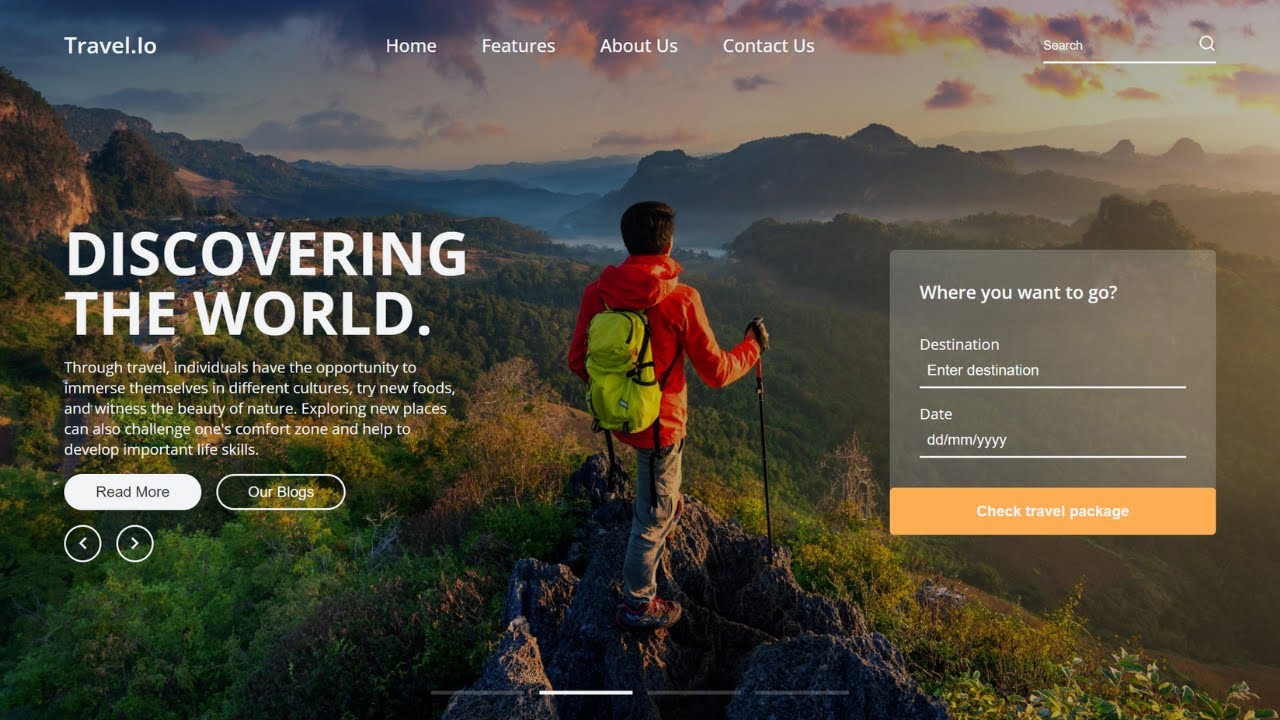This is a screenshot of a website with a full-screen background image featuring an adventurer in hiking gear. The scene is set at dusk, with the sky darkening and wisps of dark clouds adding to the atmosphere. The hiker, seen from behind, stands atop a peak adorned with shrubbery, gazing to the upper right at an awe-inspiring view of misty mountain ridges. He is wearing a red windbreaker and a yellow backpack, gray pants, and brown boots, and holding a pair of black trekking poles.

To the left of the hiker, in white font, is an inspirational text: "Discovering the world through travel. Individuals have the opportunity to immerse themselves in different cultures, try new foods, and witness the beauty of nature. Exploring new places can also challenge one's comfort zone and help develop important life skills."

Below the text are two buttons: one white with black font that says "Read More," and another transparent with white font that says "Our Blogs." Further down, there are two small circles with left and right arrows, presumably for navigating through a carousel or image gallery.